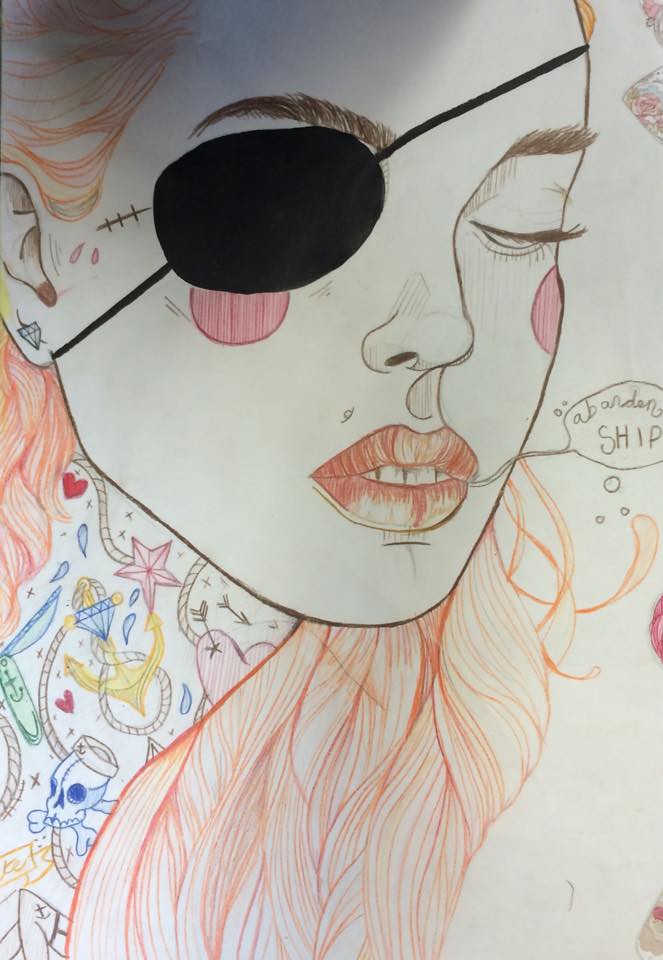The image is a detailed drawing of a female face, predominantly occupying the upper portion of the composition. The woman has striking orange hair that cascades from the upper left corner to the bottom right. Her dark brown eyebrows contrast with her almost orange lips. Notably, she bears red circles under each eye, and her right eye is covered by a black eye patch. The eye patch is secured by a strap that runs underneath her ear and across her forehead. Emanating from her mouth is a speech bubble that reads "Abandon Ship," accompanied by a few smaller bubbles. 

On the left side of the image, her neck is adorned with an array of tattoos. These include a red star, a blue skull and crossbones topped with a sailor's hat, various hearts, a yellow anchor, a blue diamond, and intricate rope designs, adding to the character's rugged and adventurous appearance.